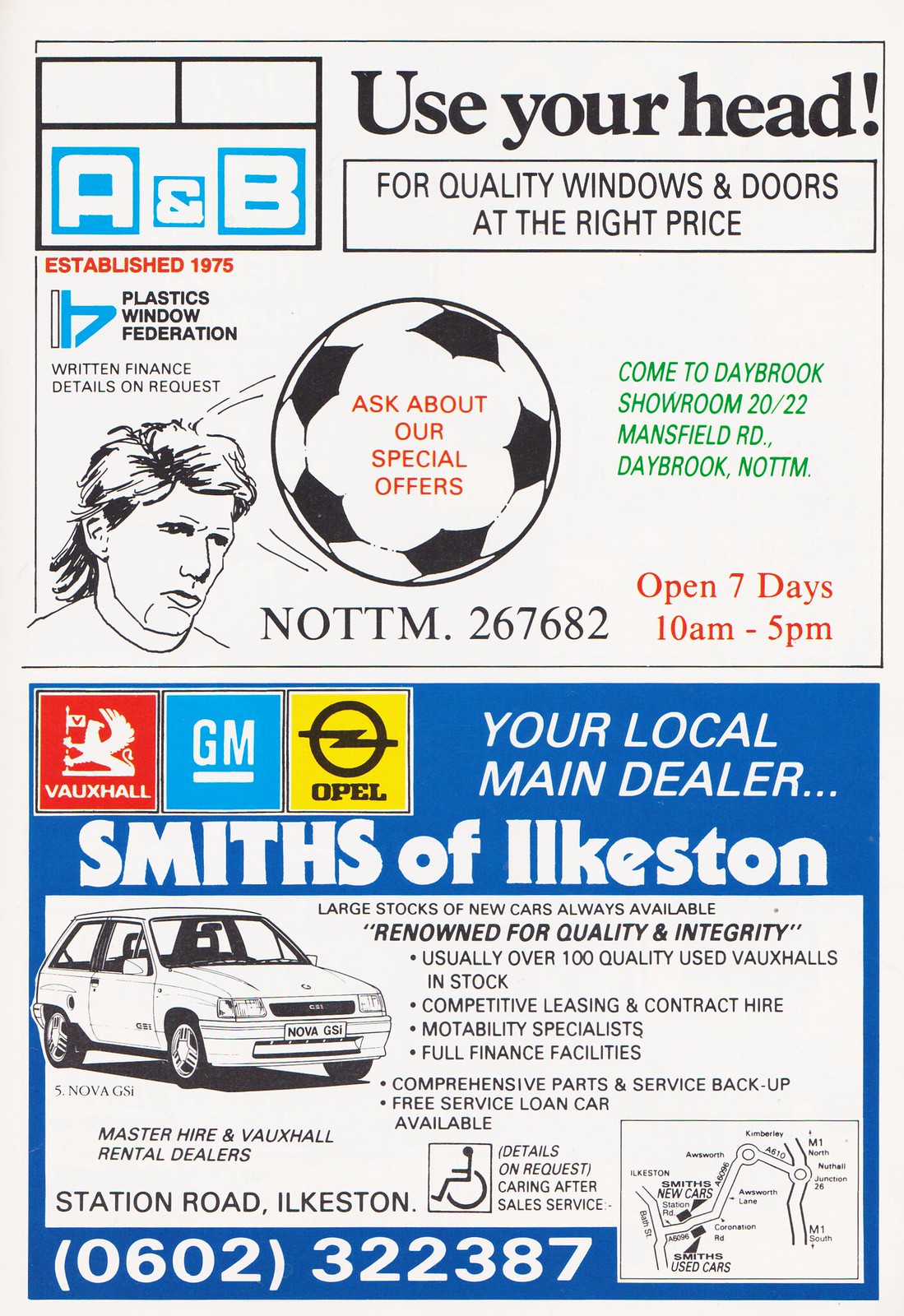The photograph displays an old British football magazine featuring two distinct advertisements. The upper half of the page advertises A and B, established in 1975, promoting quality windows and doors with the slogan "Use Your Head." The ad is visually striking with blue squares displaying the letters A and B, a red text noting its establishment year, and a large image of a man heading a soccer ball that reads "Ask About Our Special Offers." Additional details include the Plastics Window Federation mentioned in black, finance details available upon request, and their showroom address at 20-22 Mansfield Road, Daybrook, Nottingham, along with their opening hours (7 days a week, 10 am-5 pm) and contact number NOTTM 267-682.

The bottom half of the page advertises "Smiths of Ilkeston," your local main dealer, identifiable by three logos: Vauxhall, GM, and Opel. A prominent black-and-white illustration of a sedan takes center stage, accompanied by numerous bullet points detailing their services. The advertisement also features the dealership's address, contact information, and a small location map in the lower right corner to guide potential customers to the dealership.